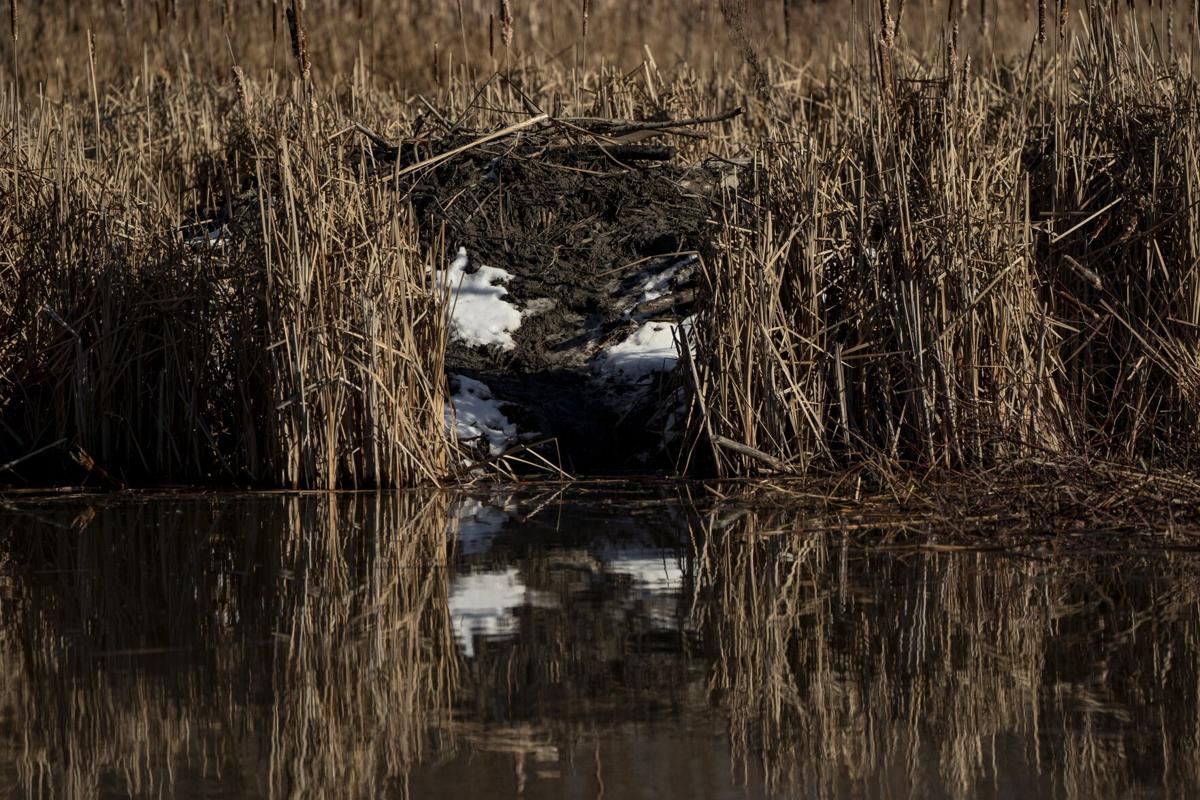This color photograph, oriented in landscape, reveals a serene yet desolate nature scene. It captures a brown, swampy pond that spans the lower half of the image, seamlessly reflecting its surroundings. The water's surface mirrors an overgrowth of light brown reeds and dried bushes lining both banks, evoking a sense of a cold winter's day. The upper center of the image features a small cave-like hole, partially covered by a shelf of dirt and patches of melting snow, both above and beside the opening. These natural elements, stark and lifeless, suggest the seasons of fall or winter. The image, devoid of animals, people, or cars, embraces the style of photographic representational realism, focusing on the raw, untouched beauty of the scene.